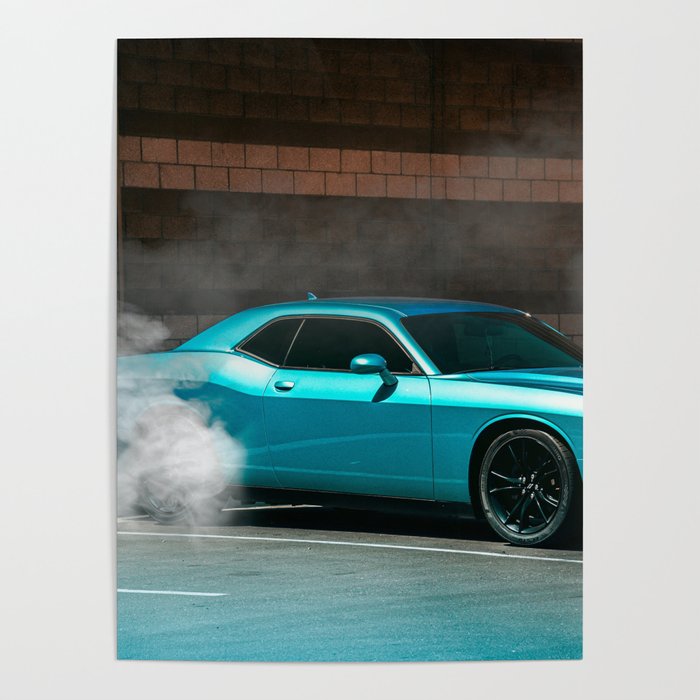In the center of the image, there is a light blue muscle car that appears to be in the midst of a high-energy burnout. The car, which exudes a pristine, almost brand-new appearance with a shiny exterior reminiscent of a Mustang, is the focal point of the scene. Its back tires are shrouded in billowing white smoke, clearly indicating that the vehicle is generating significant power as it prepares to launch forward. Surrounding the car, thin wisps of light gray smoke contrast with the denser, whiter clouds enveloping the rear wheels. Below the vehicle, the setting is a mundane parking lot, evident from the white horizontal markings on the ground. The backdrop features a brick wall with a mix of dark brown and light gray hues, adding a touch of industrial ambiance to the scene. The composition captures the raw power and excitement of the moment, with the car poised for action against the urban backdrop.